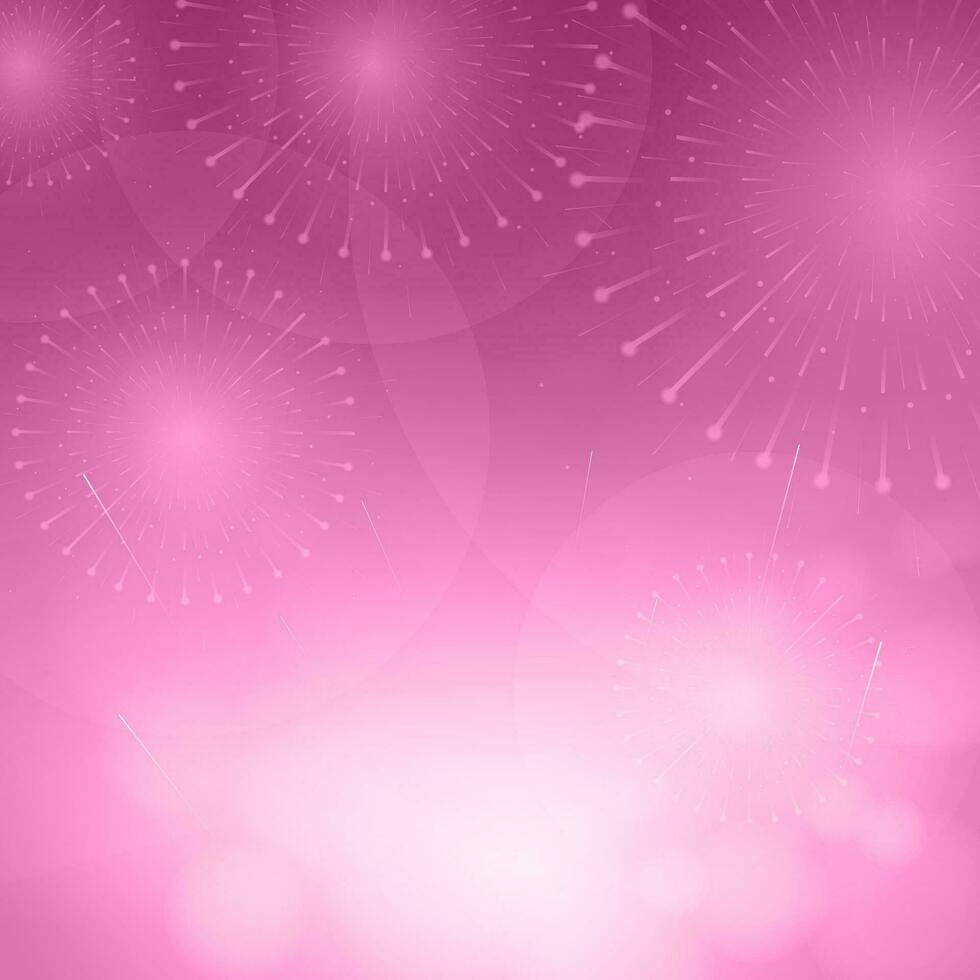This square image features a gradient of pinkish-purple hues, transitioning from a deep, rich shade at the top to a nearly white, washed-out color at the bottom, where the intensity of a bright light appears to emanate. The light source seems to be positioned behind the lower part of the image, creating an ethereal glow that gradually shifts more towards pink as it extends outward. Scattered throughout the image are several starburst-like patterns, reminiscent of tiny fireworks. These starbursts vary in size, with some being prominent and large while others are just beginning to emerge. The intricate interplay of color variations and starburst patterns adds a dynamic and mesmerizing quality to this simple yet captivating artwork.